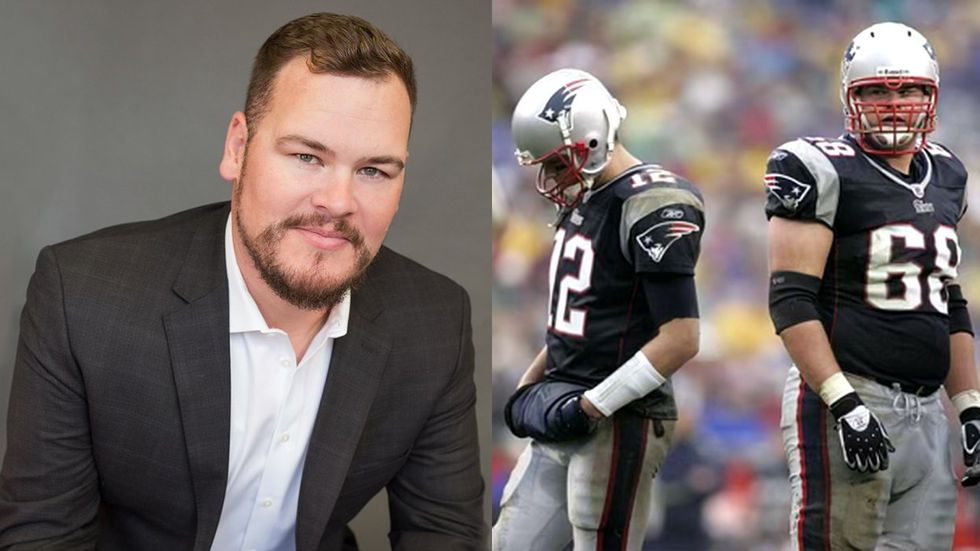This combined image features two photos side by side. On the left, there is a well-groomed young man with brown hair, a receding hairline, and a goatee beard. He has blue eyes and fair skin. He is wearing a suit jacket with a black or dark gray checker-like pattern, over a white shirt open at the collar. The right-hand image depicts two New England Patriots football players in uniform during a game. The player on the left is wearing the number 12, with a gauntlet or bandage on his left wrist. The player on the right, number 68, has the same American flag-themed helmet design. He is wearing white pants with blue stripes along the sides, black elbow pads, and gloves. The background shows a blurry stadium filled with spectators. The similarity in appearance suggests that the man in the suit in the left photo is likely the same person as the player wearing number 68 on the right.